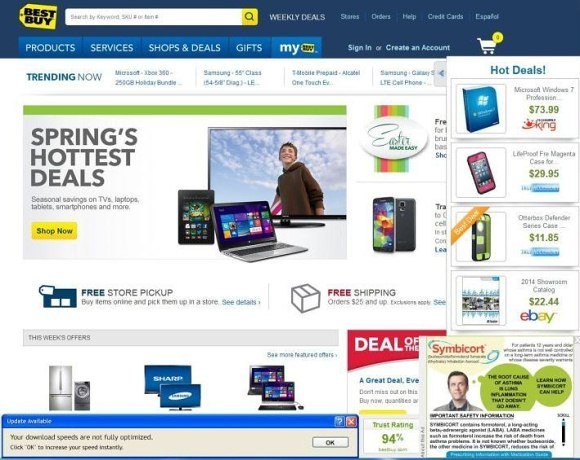This is a screenshot from the Best Buy website, showcasing its vibrant and bustling homepage. The iconic Best Buy logo, featuring bold black text on a yellow price tag resembling a sale tag, sits prominently on a blue header. Adjacent to this logo is a search field with a yellow magnifying glass button. The header also includes several navigation options: Weekly Deals, Stores, Orders, Help, Credit Cards, and an option to switch to Espanol. Below the Espanol option is a shopping cart icon indicating it is currently empty.

In the main menu, the options listed are Product Services, Shop Deals, Gifts, and My Best Buy, with additional prompts to Sign In or Create an Account. Highlighting popular items, the 'Trending Now' section features an Xbox 360 holiday bundle, a 55-inch Samsung TV, a T-Mobile prepaid plan, and a Samsung Galaxy S series phone (partially obscured).

A 'Hot Deals' panel has been expanded from the right side, displaying limited-time offers like Windows 7, a magenta phone case, and other undistinguished items, including something on eBay that's too small to discern clearly. 

To the left of the screen, a large section titled "Spring's Hottest Deals" promotes seasonal savings on TVs, laptops, tablets, smartphones, and more, accompanied by a 'Shop Now' button in yellow. A related image on the right features a tablet, a laptop, and a TV. Below this, options for free store pickup or shipping are available.

Additionally, to the right, there are a few phones listed for sale. Lastly, at the very bottom of the page, 'This Week's Offers' are highlighted, displaying a refrigerator, a washing machine, two TVs, and a couple of laptops.

Overall, the webpage appears very busy and cluttered, filled with numerous advertisements and items for sale, creating a sensory overload for the viewer.